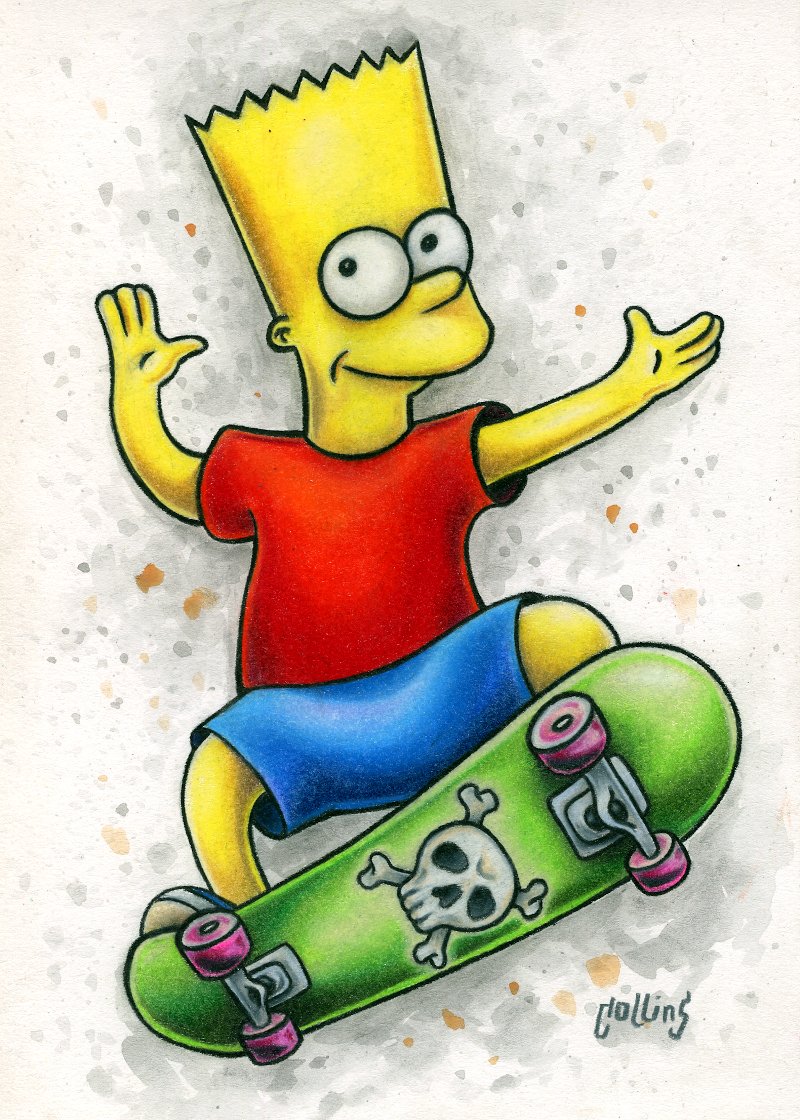This image features a yellow-skinned Bart Simpson from the iconic show "The Simpsons," recognizable by his spiky, zigzag-patterned hair and large white eyes with black pupils. Bart is depicted in mid-action, as if he's performing a skateboard trick. He wears a red short-sleeve t-shirt and blue shorts. The green skateboard with purple wheels, showing a skull and crossbones symbol on its underside, is captured tilted in the air. Bart's left arm is extended outward at shoulder height with his palm facing up, while his right arm is bent at the elbow, seemingly waving. The background is predominantly white, accented with gray specks and orange dots for decorative effect. In the bottom left corner of the image, the signature "Collins" is visible.